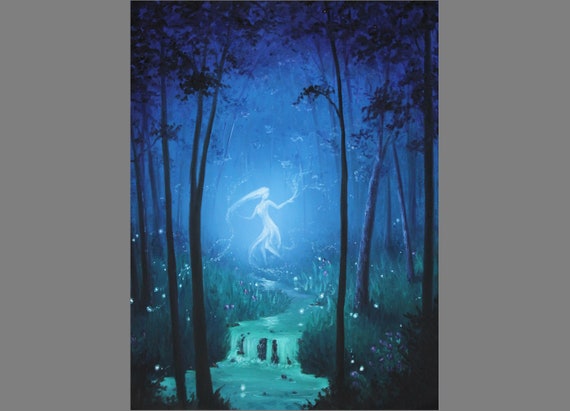In the heart of a mystical, blue-hued forest, a luminous woman exudes an ethereal glow, commanding the scene. Dressed in a flowing gown with frills, she stands along a milky, stream-like river that courses through the forest. Tall trees with leafy crowns rise around her, their green grass base adorned with white, glowing flowers. The night scene is filled with an array of fireflies and has an overall fantasy ambiance, emphasizing her otherworldly presence. The woman's long hair flows gracefully behind her, further enhancing her magical and ghostly appearance. Despite the enchanting details of the setting, she remains the central light source, illuminating the surreal, digitally illustrated landscape. The image is framed with a grey background on either side, adding to the focus on this captivating, fairy tale-like tableau.